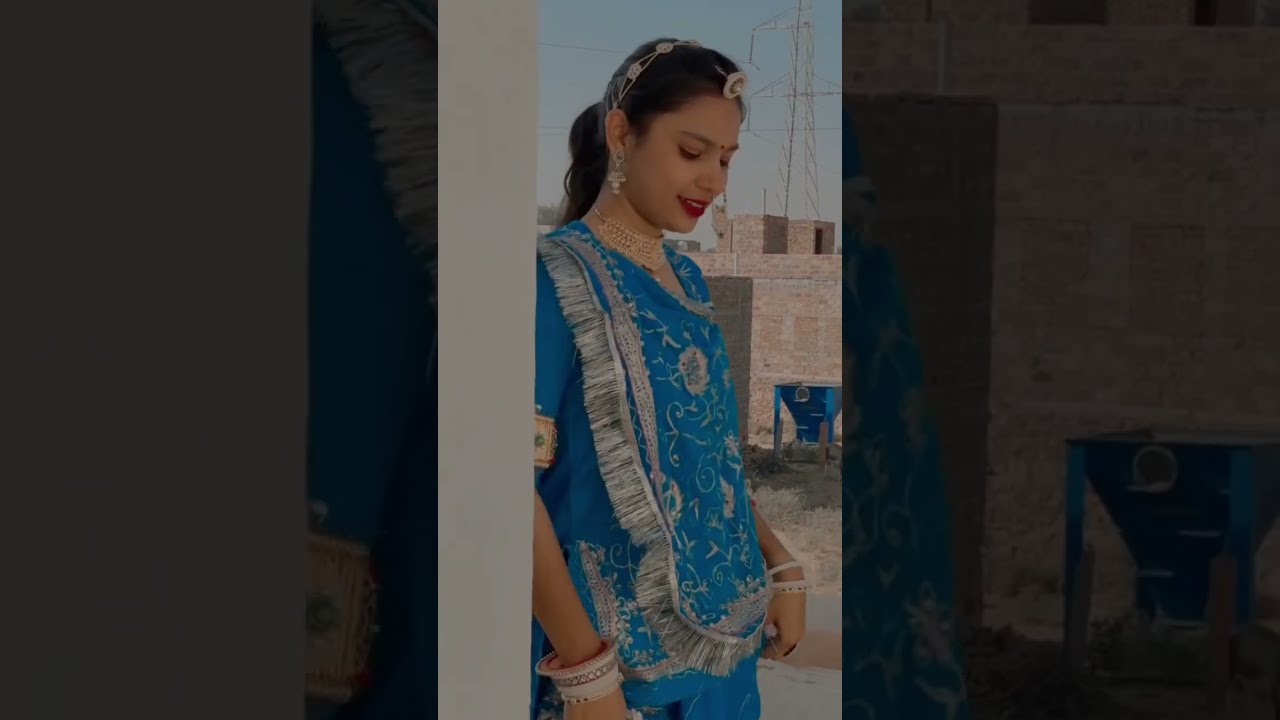This photograph, taken with a smartphone camera in a vertical orientation, features a young Indian woman dressed in a traditional deep blue sari adorned with ornate silver fringing and intricate floral patterns. Central to her attire is a beige medallion accentuated with blue-green filigree. Her ensemble is complemented by an array of jewelry, including bracelets on both wrists, dangling earrings, a choker-style golden necklace, and a traditional hair ornament that cascades along her hairline, which is pulled back into a ponytail secured with a ribbon. The woman, with a serene expression and adorned in red lipstick, is looking downwards, her face calm and composed. She stands outdoors against a beige brick or adobe industrial building, which features a blue construction equipment piece, likely a cement mixer, on its right side. A cell phone or radio tower is visible over her left shoulder, extending upwards into a cloudless, muted blue sky. The image, slightly dull and possibly filtered, is framed by darkened rectangles on either side, suggesting it was viewed through a wall or door.